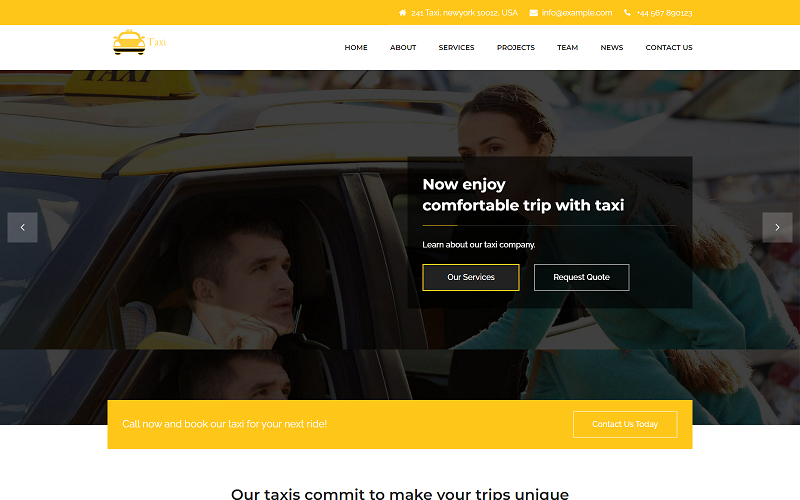The image depicts the homepage of a New York-based taxi company’s website. At the top of the site is a prominent yellow bar with white text, displaying a home icon followed by "241 Taxi, New York, 10012, USA." Next to this is an envelope icon with "info" and a phone number. Below the yellow bar is a white navigation strip with a list of clickable sections: Home, About, Services, Projects, Team, News, and Contact Us.

On the left side of this navigation strip, there is an image of a yellow taxi facing forward. The image below this navigation area is a wide, rectangular photo with a dark, somewhat grayed-out filter. It portrays a close-up of a taxi with the driver, positioned on the left looking towards a woman who is standing outside the car. The woman, who has dark hair, is leaning slightly towards the taxi and engaging in conversation with the driver.

Above the woman is a black rectangular box containing the text: "Now enjoy a comfortable trip with Taxi. Learn more about our taxi company." Additionally, there is a yellow-highlighted box reading "Our Services." At the bottom of the page, there is a statement: "Our taxis commit to making your trips unique." The overall design and imagery convey a professional and user-friendly interface aimed at promoting the taxi services.